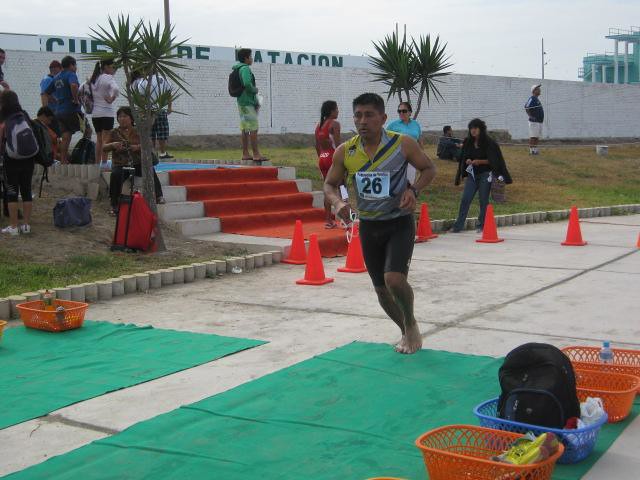In the image, a man, likely of Hispanic descent, is poised to start running, suggesting he's about to participate in a track and field event. He wears black sprinting shorts that go above the knee and a yellow, green, and light gray striped sleeveless jersey. A white sign with the number 26 is pinned to his chest. The man has short black hair and appears to be in his early 30s. He stands on a green mat laid over a stone or concrete ground, situated center frame of the photograph.

Surrounding him, the scene features several distinct elements. Immediately behind him, there are six orange pylons. To the left, a set of concrete steps covered in red carpeting ascends, with a group of onlookers standing nearby. The background reveals a grassy hill and a white wall running along the entire length of the image. On the lower left side of the picture, there are three orange baskets and one blue basket, one of which contains a black book bag. Additional items like rugs, more baskets, and book bags lie scattered around the stone flooring. The photograph is taken outdoors, likely in the middle of the day, with colors vividly represented as orange, gray, green, tan, black, blue, and red.